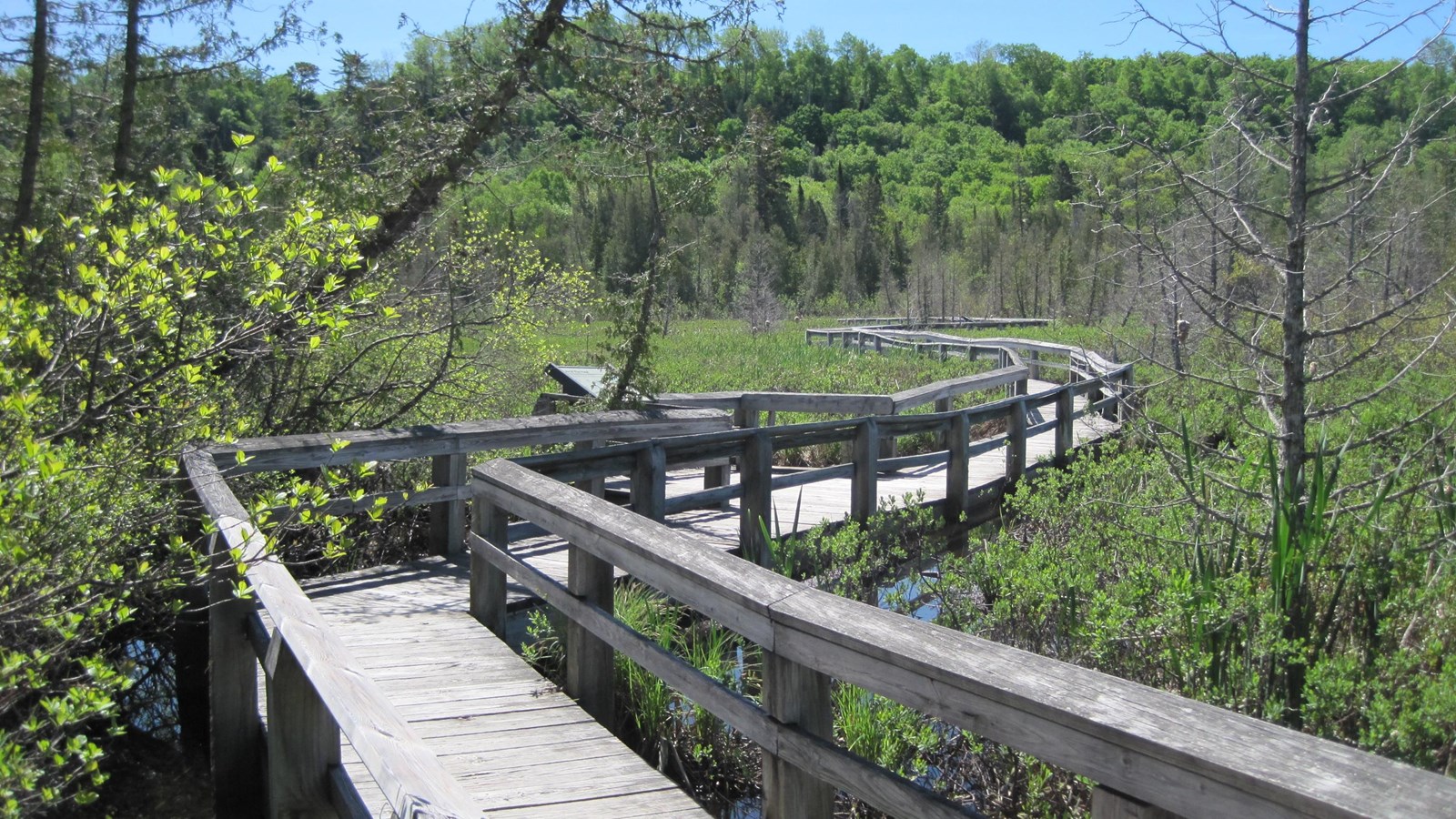The photograph captures a scenic view of a long wooden walkway stretching through a serene swamp environment, reminiscent of the Everglades. The light brown, weathered-gray walkway curves in a zigzag fashion and is wide enough for two people to walk side by side. It features sturdy railings on both sides, providing safety and a place for pedestrians to rest their arms. A few feet from the camera, the walkway broadens into a viewing area that includes an information placard attached to the railing. On either side of the walkway, a small body of water, likely part of a lake or swamp, shimmers under the sunlight. This water area is surrounded by lush green trees and bushes, which further extend into the distance, creating a dense forest canopy. The sky above is clear and vividly blue, adding a tranquil backdrop to the verdant scene.